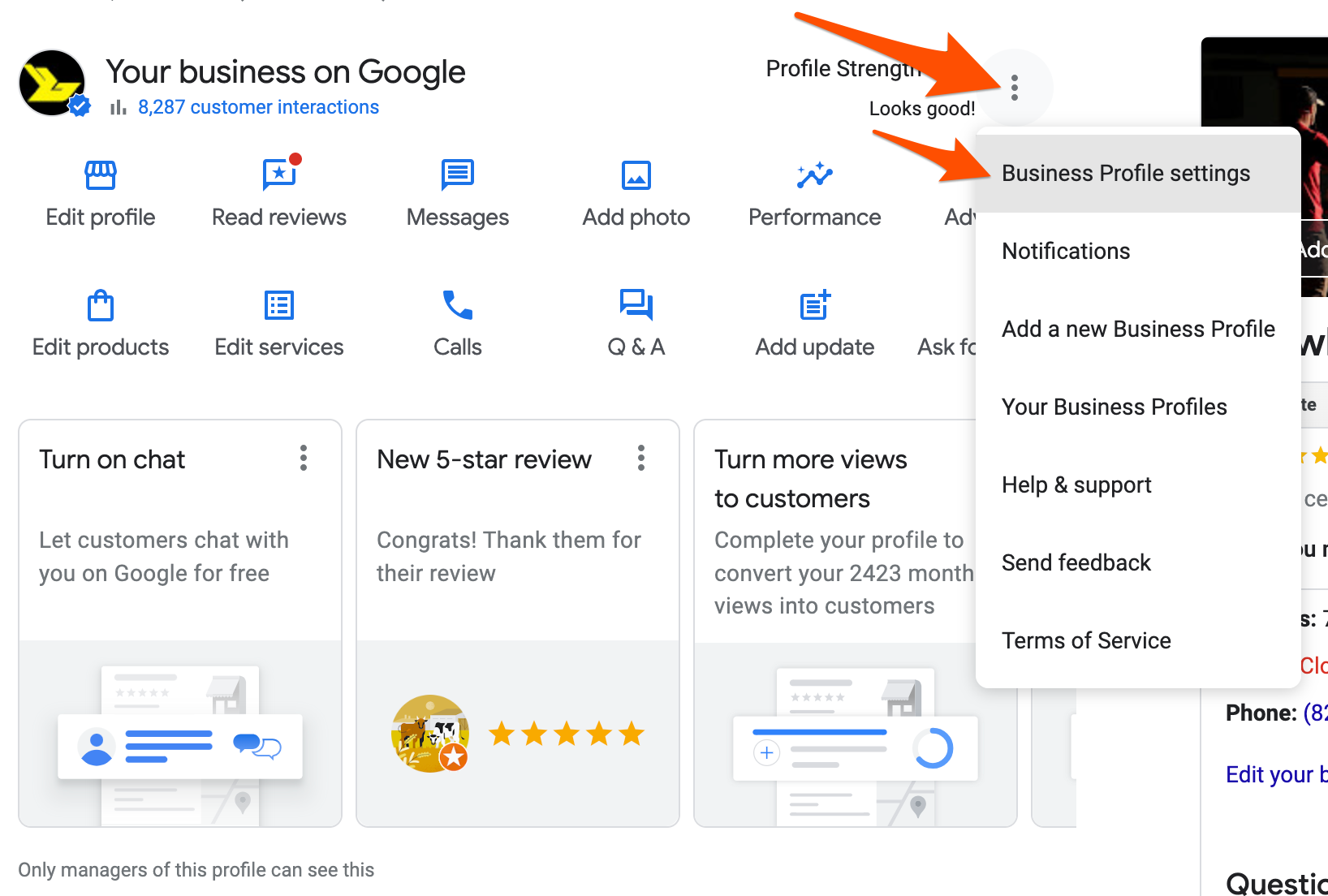This image features an advertisement for a downloadable app with a white background. The ad demonstrates various functionalities of the app designed to help users manage their business presence on Google. 

On the left side, in bold black lettering, it reads "Your business on Google," followed by a statistic in blue lettering stating "8,287 customer interactions."

On the right side, the text reads "Profile Strength: Looks Good," accompanied by a settings icon represented by three vertical dots. Clicking this icon reveals a drop-down menu with options including: 
- Business Profile Settings
- Notifications
- Add a New Business Profile
- Your Business Profiles
- Help and Support
- Send Feedback
- Terms of Service

The main section of the ad showcases several clickable links for managing the business profile:
- Edit Profile
- Read Reviews
- Messages
- Add Photo
- Performance
- Edit Products
- Edit Services
- Calls
- Q&A
- Add Update

Two additional links are partially obscured by the drop-down menu.

At the bottom of the page, several prompts are highlighted:
- "Turn on Chat: Let customers chat with you on Google for free."
- "New 5-Star Review: Congrats! Thank them for their review."
- "Turn More Views Into Customers: Complete your profile to convert your 2,423 monthly views into customers."

In the bottom left corner, a note in blue lettering reads, "Only managers of this profile can see this."